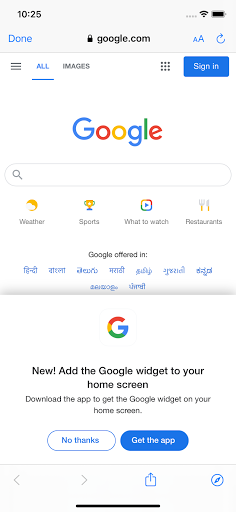This is a screenshot capturing a Google search results page. 

At the top of the image, there is a gray background with some text that reads "1025." To the right, there are some gray dots, a black Wi-Fi symbol, and a black battery icon. Just below, a blue button is labeled "Done."

The URL bar displays "google.com" along with a padlock icon, indicating a secure connection. Below this, blue icons including an "A" and an arrow are visible.

The main body of the page has a white background with various elements:
- A gray search bar with a magnifying glass icon.
- The Google logo in blue, red, yellow, and green.
- A "Sign in" button inside a blue and white box.

Beneath these elements, several search category options are listed:
- "Weather" with a gold and white cloud and sun icon.
- "Sports" with a gold and blue trophy icon.
- "What to watch" with a multicolored box in red, gold, green, and blue.
- "Restaurants" with a gray and gold fork and knife icon.

Further down, it says "Google offered in" followed by various language symbols in blue.

At the bottom of the screen, there is a prompt with the Google "G" logo inviting users to "Add the Google widget to your home screen," along with directions to download the app. There are two blue and white boxes for user options: "No thanks" and "Get the app," with "Get the app" currently selected.

Finally, a gray navigation bar at the bottom features a back arrow, a forward arrow, a share icon, and a compass-like icon, with a black line below these icons.